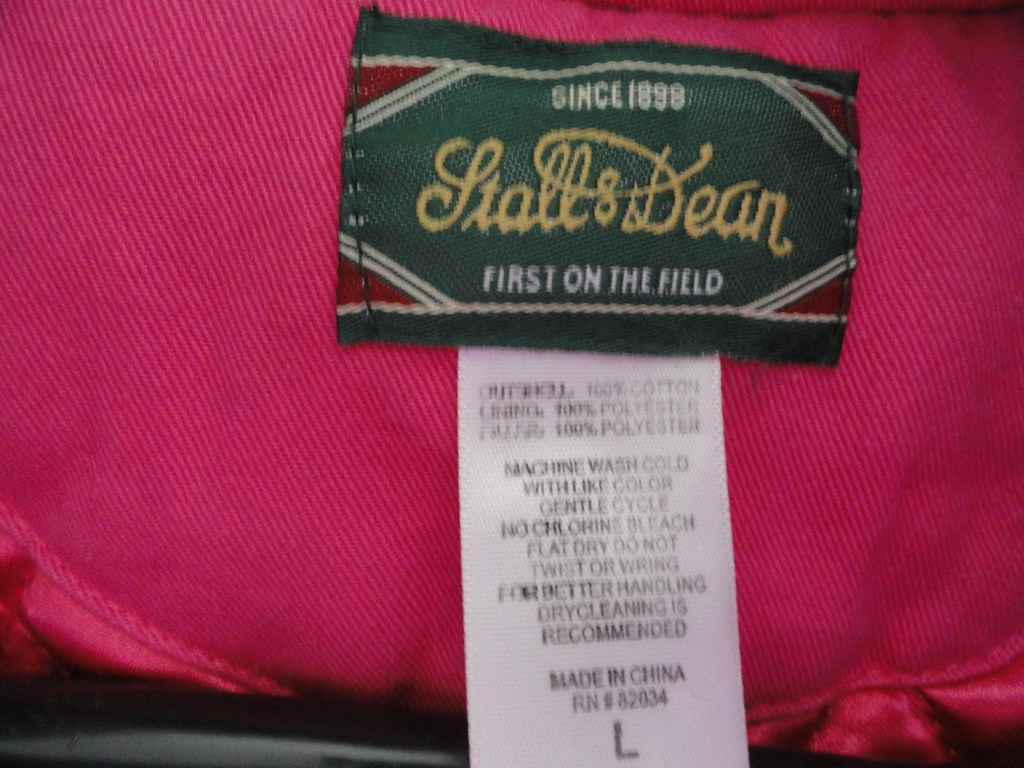Here is the cleaned-up and detailed caption:

"A detailed close-up of a garment tag, likely from a jacket made of canvas or denim material. The main tag is black with a prominent white rectangle outlined at the top and bottom, with maroon triangles marking each corner. Below the upper white line, the text 'Since 1898' is centered. In yellow cursive script, the brand name 'Stahls & Dean' is displayed in the middle. Underneath, the phrase 'First on the Field' is written in white text. The bottom of the main tag is bordered by another white line. Attached to this is a smaller white care tag that reads:

- Shell: 100% Cotton
- Lining: 100% Polyester
- Filling: 100% Polyester

Care instructions specify to machine wash cold with like colors on a gentle cycle, avoid chlorine bleach, dry flat, and do not twist or wring. It also recommends dry cleaning for better handling. The tag indicates the garment is 'Made in China' with an RN number: 82034NL."